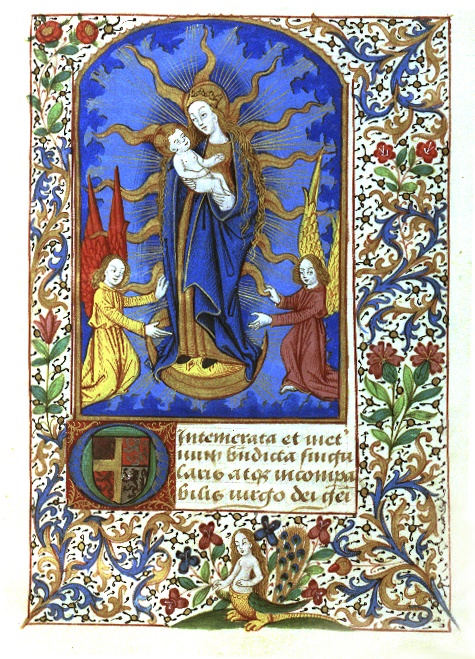This image is a stunning stained glass window featuring a central figure of a woman with long brown hair, dressed in a royal blue robe over a golden dress. She stands on what appears to be a pedestal, holding a naked infant with brownish hair. Radiating from behind the woman are sun rays, giving her an almost divine aura. Flanking her are two children with wings: one on her left has red wings and wears a red dress, while the one on her right has golden wings and is clad in a gold dress. The blue background accentuates the figures.

Surrounding the central scene, the outer edges of the window are adorned with vibrant red flowers, green leaves, and stems, interspersed with swirling lines of blue and gold. There are also splotches of color—deep red, green, gold, and blue—scattered throughout, adding to the window's intricate design. At the bottom of the window, under this elaborate scene, is a mystical mermaid-like creature with dragon feet and a peacock tail, completing the composition. The base of the window bears some unreadable goldish-brown text, adding a mysterious element to this already detailed and vivid depiction.